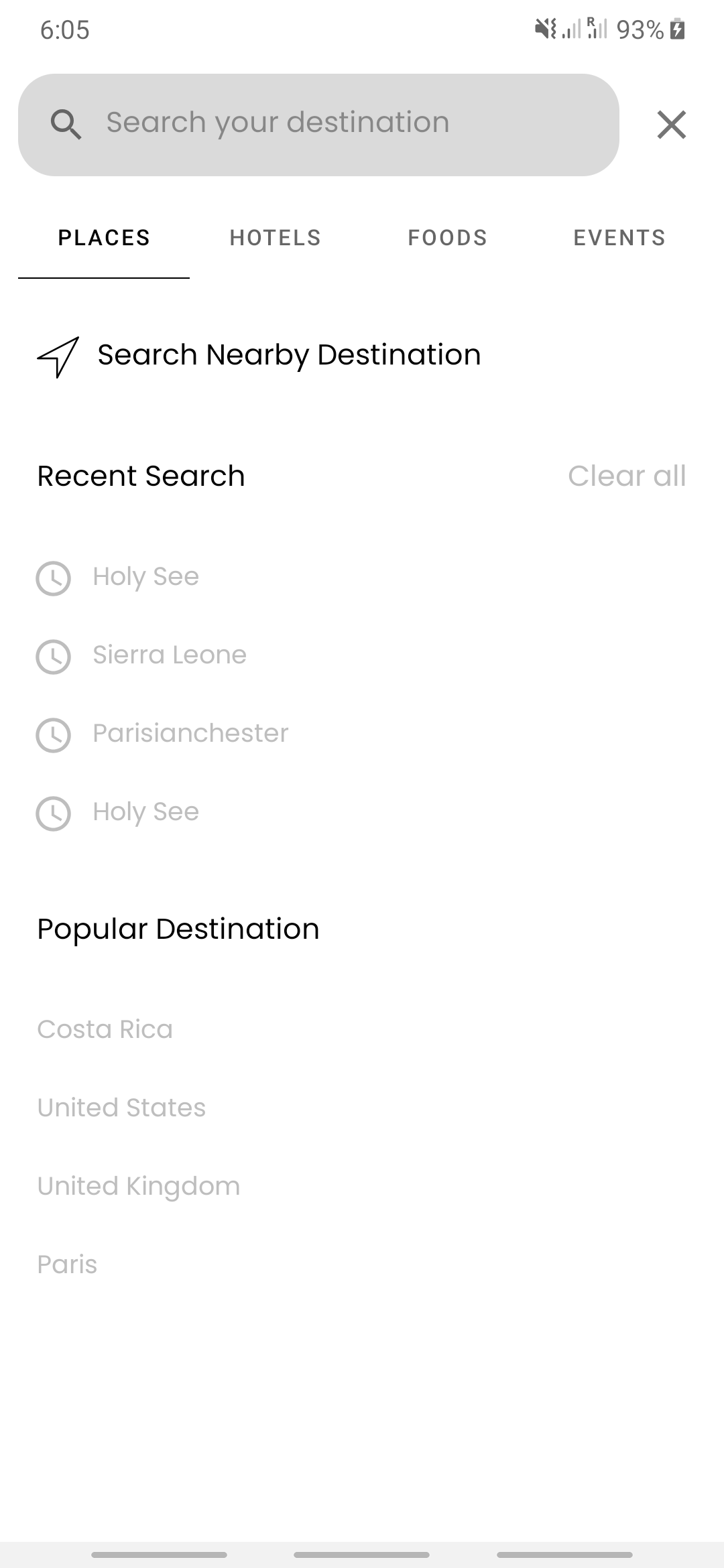The image is a screenshot with a solid white background. In the upper left corner, black text displays the time as 6:05. The upper right corner shows that the speaker is off, and the battery is at 93%. Below that, there is a gray search box with faint gray text that reads "Search your destination."

Directly underneath this search box, there are five labeled icons from left to right: Places, Hotels, Foods, Events. Below these icons, there's another section titled "Search nearby destinations."

Further down, the category "Recent Search" is listed, with entries for "Holy See, Sierra Leone, Parisian Chester, Holy See". To the upper right of the words "Recent Search," there is an option to "Clear All" in light gray text.

At the bottom left, "Popular Destination" is listed in black text. Under this heading, light gray text lists "Costa Rica, United States, United Kingdom," with "Paris" mentioned last.